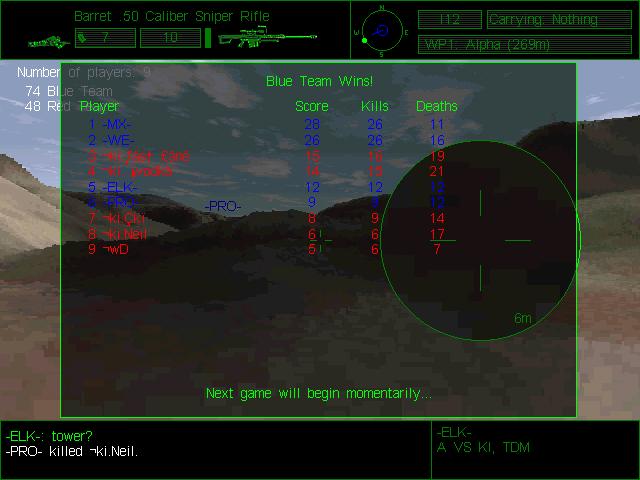The image is a screenshot from an older first-person shooter video game, appearing to be more than 20 years old. The screen has distinct black borders at the top and bottom. In the center, there's a transparent black rectangle with green edges. Below it, a notification reads, "Next game will begin momentarily." The lower-left corner displays the text "elk... tower?" in green, with "pro-killed-ki.neil" in white below it. The lower-right corner has additional green text: "ELK-AVSKI, T-O-M." Along the top, "Barrett 50 caliber sniper rifle" is written, and a picture of a person lying down and holding a gun is visible. The desert-like landscape showcases sandy terrain and distant mountains, under a blue sky with some clouds. The interface also includes various measurements and scores, indicating a detailed HUD. Notably, a compass and team stats—"Blue Team Wins" with associated player counts (974 for blue, 48 for red)—are part of the game display.